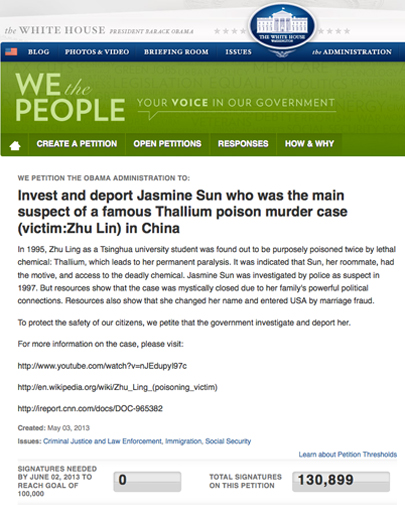The image showcases a detailed graphic layout of a petition platform associated with the White House during President Barack Obama's administration. At the top, the White House emblem is prominently displayed, featuring an illustration of the iconic building set against a white background, alongside President Barack Obama's name. An American flag is situated in the corner, accompanied by a menu listing the following categories: "Blog," "Photos and Video," "Briefing Room," "Issues," and "The Administration."

Beneath this header, a green rectangular banner carries the title, "We the People: Your Voice in Our Government," outlining various options such as "Create a Petition," "Open Petitions," "Responses," and "How and Why." The gray text in this section reads, "We petitioned the Obama administration to," followed by a bolded statement in black text: "Invest and deport Jasmine Sun, who was the main suspect of a famous thallium poison murder case, victim Zhulian in China."

At the bottom of the graphic, there is a call to action indicating the need for signatures. It states, "Signatures needed by June 2, 2013 to reach goal of 100,000." Beside this, a square shows the number zero. To the right, it lists the "Total Signatures on this Petition," with a corresponding square that displays the number 130,899.